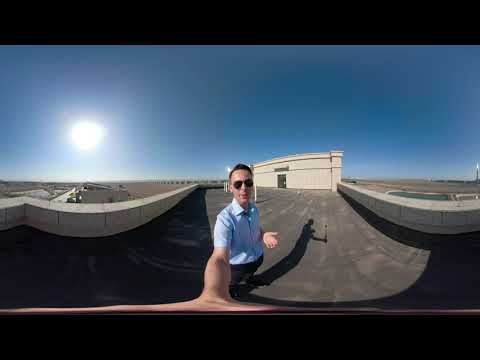This horizontally-aligned rectangular image features a man positioned centrally, wearing dark sunglasses and a light blue short-sleeve button-down collared shirt along with black pants. The man has short brown hair and a fair complexion. His left hand is held close to his body with the palm facing upwards, whereas his right hand is outstretched towards the camera, appearing distorted and spread out along the bottom of the picture, likely due to a wide-angle or 360-degree surrounding view. The man is standing on a gray concrete surface, which might be the roof of an industrial or office building, suggesting he is at some height, potentially in a parking garage. In the background, a white stone rectangular building with a single door in the middle and no windows is visible. Flanking the image are gray stone walls. The sky above is clear blue with no clouds, and the sun is positioned in the upper left portion, indicating it is close to sunrise or sunset. Thick black borders at the top and bottom frame the image.